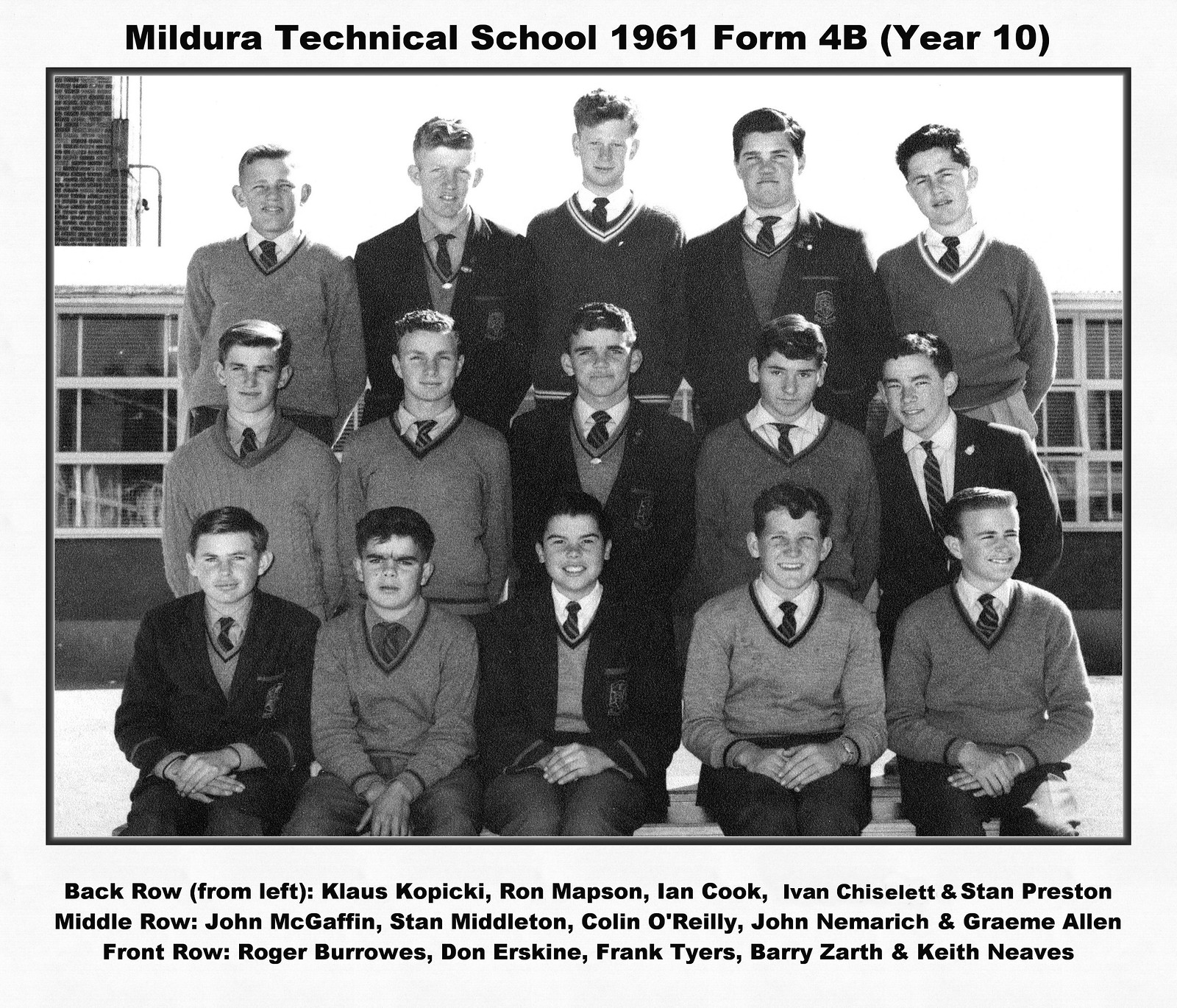The black-and-white image captures a formal class photograph from Mildura Technical School, dated 1961, and features Form 4B, Year 10 students. The picture is neatly arranged with three rows of young men: the back row has five standing boys, the middle row has five kneeling, and the front row has five sitting on the ground. These boys, appearing to be in their teenage years, are dressed in V-neck sweaters over white button-down shirts, complemented by striped ties. They also sport close-cropped hairstyles typical of the 1960s, with some styling their hair parted or combed back. A range of expressions, from smiles to serious looks, can be seen.

At the top of the photograph, the text reads: "Mildura Technical School, 1961 Form 4B, Year 10." Below the image, the names of the students are listed according to their rows: 

- Back row (from left): Klaus Kopicki, Ron Mapson, Ian Cook, Ivan Chislett, and Stan Preston.
- Middle row: John McGaffin, Stan Middleton, Colin O'Reilly, John Nemerich, and Graham Allen.
- Front row: Roger Burrows, Don Erskine, Frank Tyers, Barry Zarth, and Keith Neves.